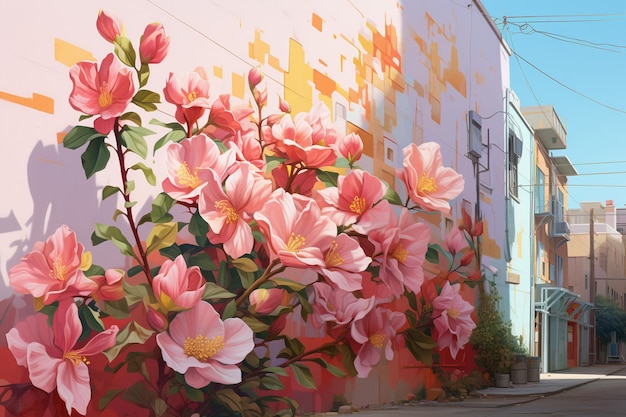This image is a detailed depiction of an outdoor scene featuring an impressive piece of wall art on a row of two-story homes. The buildings dominate the left side of the image and gradually narrow as they recede into the distance on the right. The primary focal point is the large wall with a distinct light pink tone, subtly revealing yellow and orange hues where bits of the exterior have chipped away. Covering this wall is a striking, almost three-dimensional painting of a bush with tall, reddish-brown stems and elliptical green leaves. The bush is adorned with large, vivid pink flowers, each comprising five petals with yellow centers, creating a vibrant contrast against the background. On the right side of the image, additional buildings painted in blue, orange, and off-white are visible, contributing to the lively urban palette. The sky in the upper right corner is a bright blue, crisscrossed with numerous power lines, while the lower right corner shows a sidewalk adjoining a bare street. Additional elements include garbage cans and a streetlight, enhancing the urban atmosphere. The artist has skillfully painted shadows to enhance the illusion of depth, making parts of the artwork appear as if they are popping off the wall, creating a mesmerizing optical illusion.